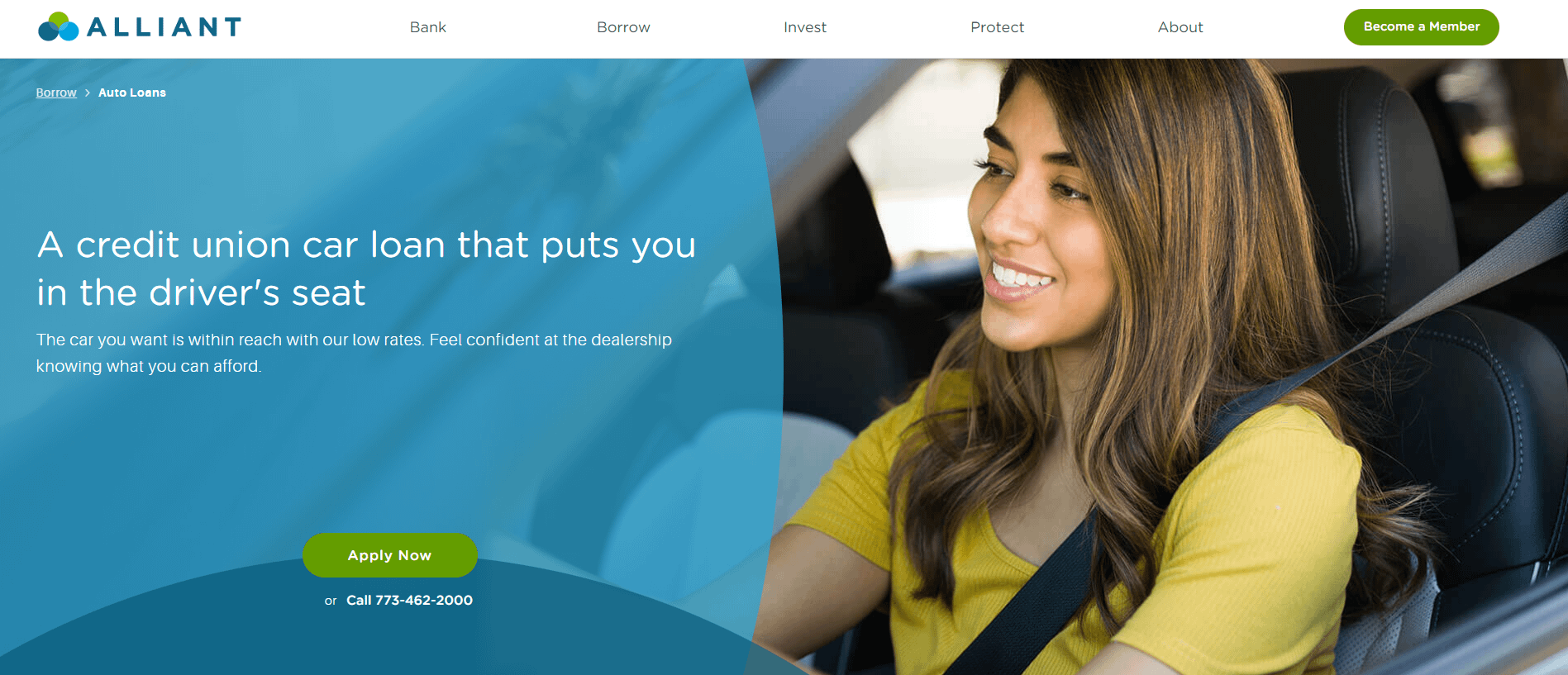The image is a promotional screenshot for Alliant, a car loan company. At the top of the screen is a white banner with navigational menu items in a dark font, reading from left to right: Bank, Borrow, Invest, Protect, About. In the upper right-hand corner, there is a rounded rectangular button shaded in green with white text that reads "Become a Member."

Below the white banner, the left side of the screen features a blue curved design in two shades of blue, partially transparent. On the right side of the screen is an image of a woman with long, dark hair, sitting inside a vehicle and looking to her left. She is wearing a seatbelt, and the perspective of the image is as if taken from outside the driver's side window. The woman is smiling, showing her white teeth, and has dark eyes, eyebrows, and eyelashes.

In the upper left corner of the image, the company's name, "Alliant," is written in all capital letters with a three-part logo in light green, dark green, and blue situated to the left of the name. 

On the blue portion of the screen, at the very top, the white font reads "Borrow -> Auto Loans," with "Auto Loans" in bold. Larger text below states, "A credit union car loan that puts you in the driver's seat," also in white. Further down in smaller white font, it says, "The car you want is within reach with our low rates. Feel confident at the dealership knowing what you can afford." At the bottom of the blue graphic section is another rounded green rectangular button with white text reading "Apply Now," followed by the contact number, "Call 773-462-2000" in white font.